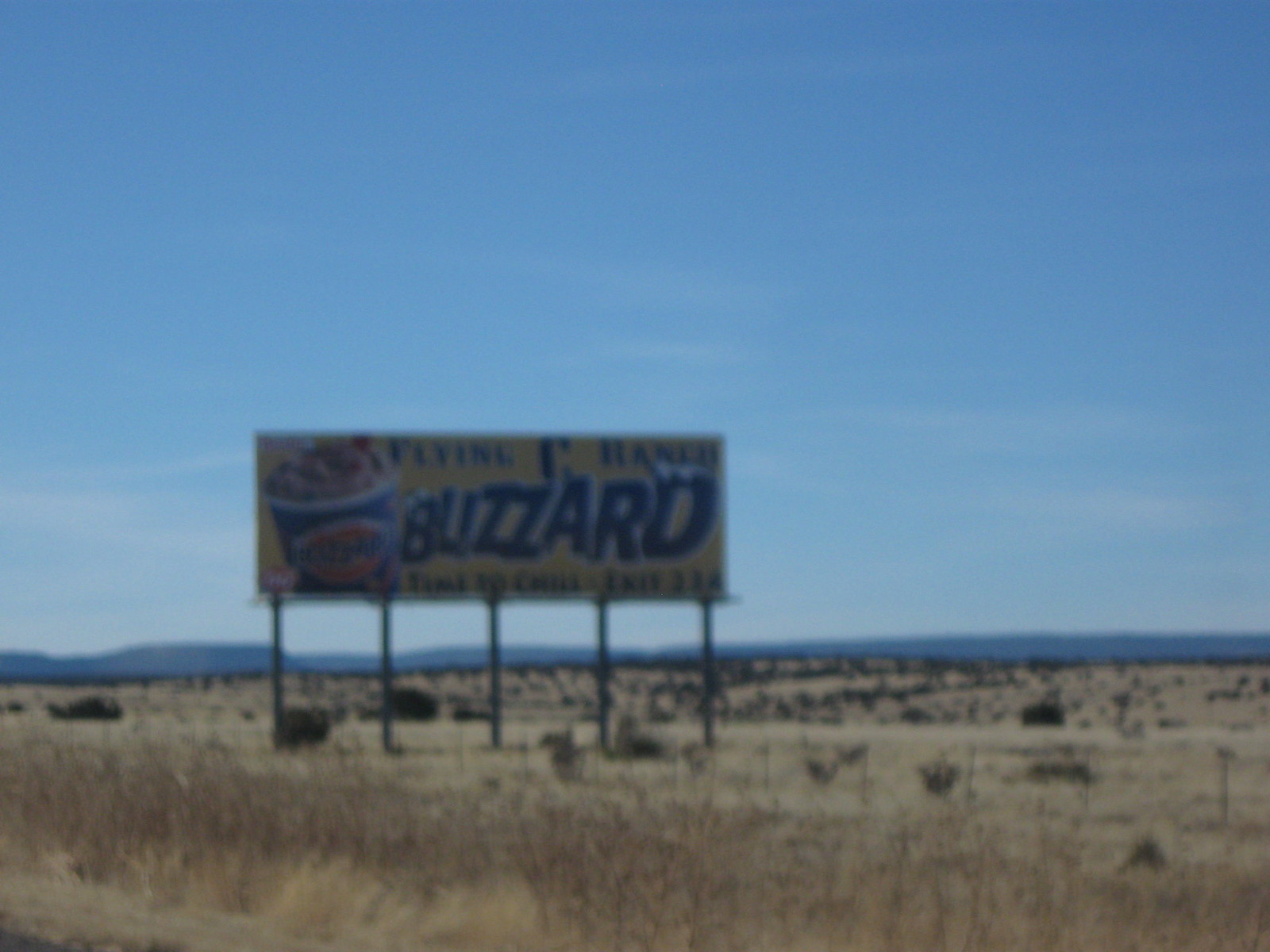A blurry, out-of-focus photograph likely taken from a roadside in a desert environment. The image features distant bluish hills beneath a clear blue sky with sparse clouds. The foreground is dominated by dry, scrubby vegetation and weeds. A prominent billboard appears in the scene, advertising a "Blizzard," reminiscent of the Dairy Queen treat. The vintage color scheme and font of the billboard suggest an older era, adding a nostalgic touch to the arid landscape.